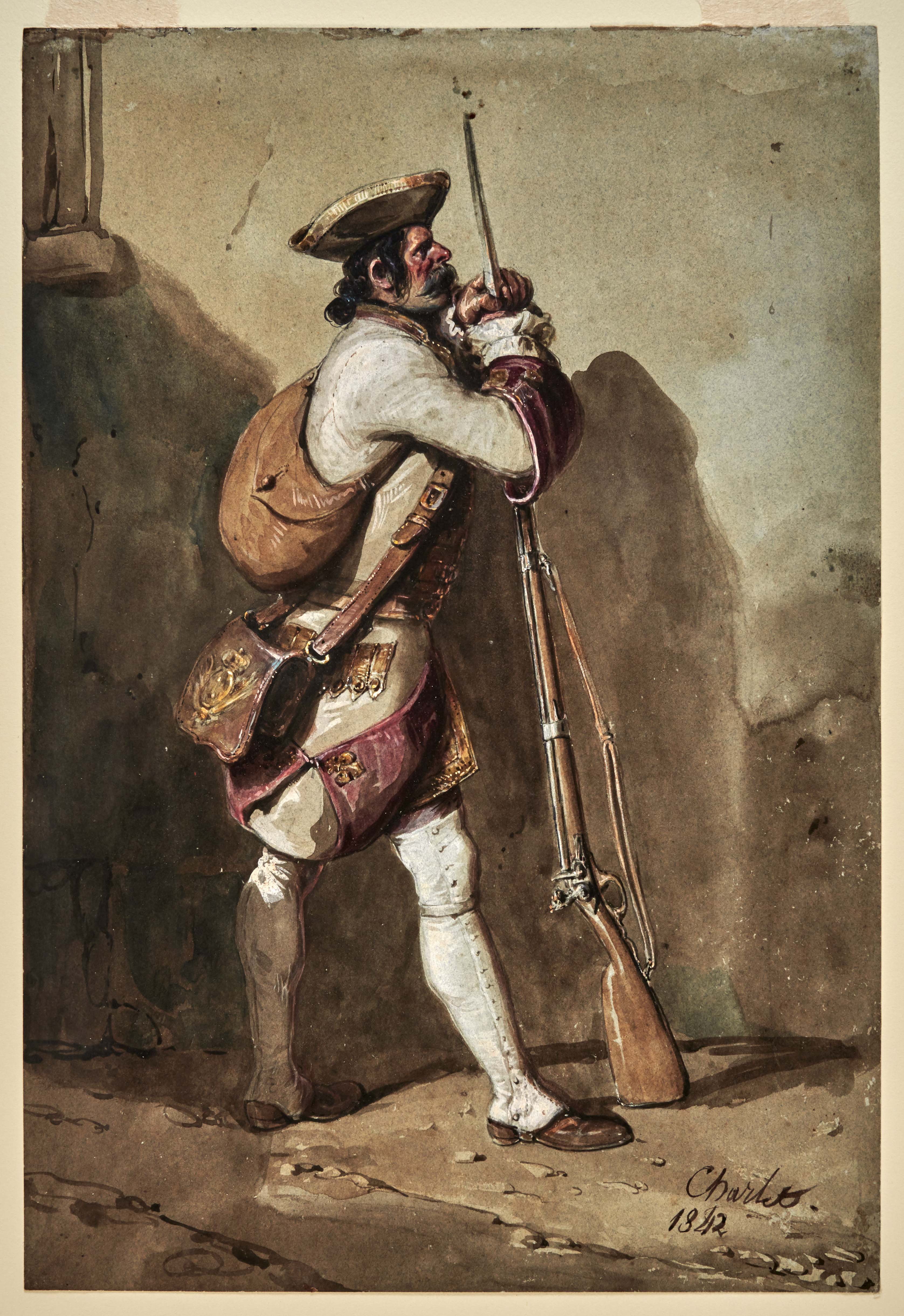The image seems to be an old photograph or postcard with a rectangular, vertical orientation and a distinctive brown-tan coloring typical of aged photos. The scene depicts a man standing sideways, looking to the right. He is adorned in long white leggings, possibly part of a white and maroon uniform, and wears a wide-brimmed, humorous brown hat atop his head, from which long brown-black hair tied in a ponytail extends. The man sports a mustache and a bright red nose.

He is carrying multiple bags—one slung over his shoulder and another, longer one draped across his body. His footwear consists of long white socks and brown shoes. The man is grasping a long musket or bayonet, which stands taller than he does. He holds the spear-like tip of the bayonet, resting its butt on the ground before him.

In the background, there is a building or a wall constructed from smooth stone, suggesting an old historical setting, possibly around the 1840s. The overall scene conveys a sense of antiquity, with the man posed as if in contemplation or readiness, against the timeless backdrop.